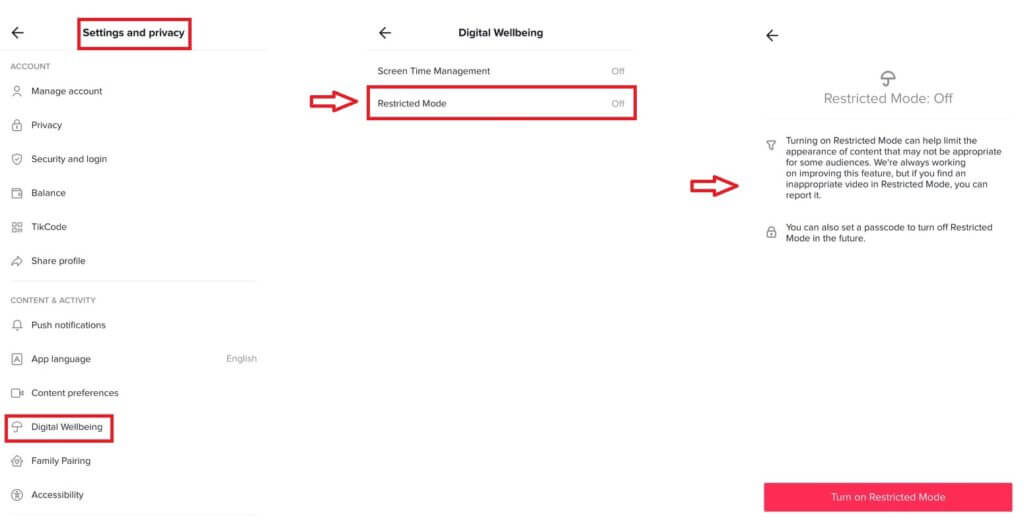This detailed image showcases a section from the Windows settings interface, specifically focusing on digital wellbeing features. The image predominantly features black text on a white background, accented with red boxes and arrows for emphasis.

At the top center, the title "Digital Wellbeing" is displayed. On the left side of the image, a menu column lists various settings options, including:
- Settings and Privacy
- Manage My Account
- Privacy
- Security
- Login and Balance
- TikCode
- Share Profile
- Push Notifications
- App Language
- Content Preferences
- Digital Wellbeing (highlighted with a red box)

Both "Settings and Privacy" and "Digital Wellbeing" are marked by red outlines. Above this menu, there's an option for "Family Pairing" and "Accessibility," with the app language set to English.

Focusing on the "Digital Wellbeing" section, the main content area describes features like "Screen Time Management Control" and "Restricted Mode." A red-outlined box surrounds this section, with a red arrow pointing to it.

On the right side, another column features a black text at the top alongside an umbrella icon. This text explains "Restricted Mode" is currently off and states, "Turning on restricted mode can help limit the appearance of content that might not be appropriate to some audiences. We are always working on improving this feature but if you find an inappropriate video in restricted mode, you can report it. You could also set a passcode to turn off restricted mode in the future."

At the bottom right corner, a prominent red box contains white text that reads "Turn On Restricted Mode."

The image clearly aims to guide users through enabling Restricted Mode to enhance digital wellbeing by limiting inappropriate content.